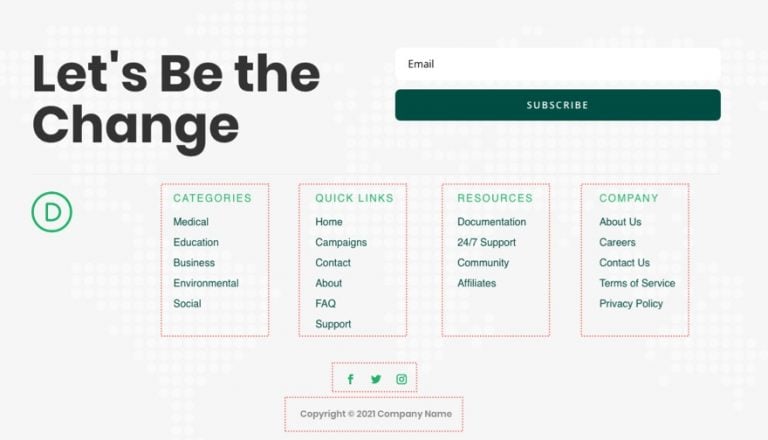The website appears to be a self-help resource, designed to encourage personal growth and positive change. In the upper left corner, a prominent phrase "Let's be the change" is displayed in large black font. Adjacent to this phrase is a white rectangular subscription box outlined with a thin green line; the word "email" is inscribed in small green font on one side, prompting users to input their email addresses. Beneath this box is a green rectangular "Subscribe" button with the text "subscribe" written in white font.

Below the subscription section, the website features four vertical rectangles presenting various categories of information. The first rectangle is labeled "Categories," followed by "Quick Links," "Resources," and "Company." Each rectangle contains a list of hyperlinks under these headings, allowing users to navigate the different sections and resources offered by the website.